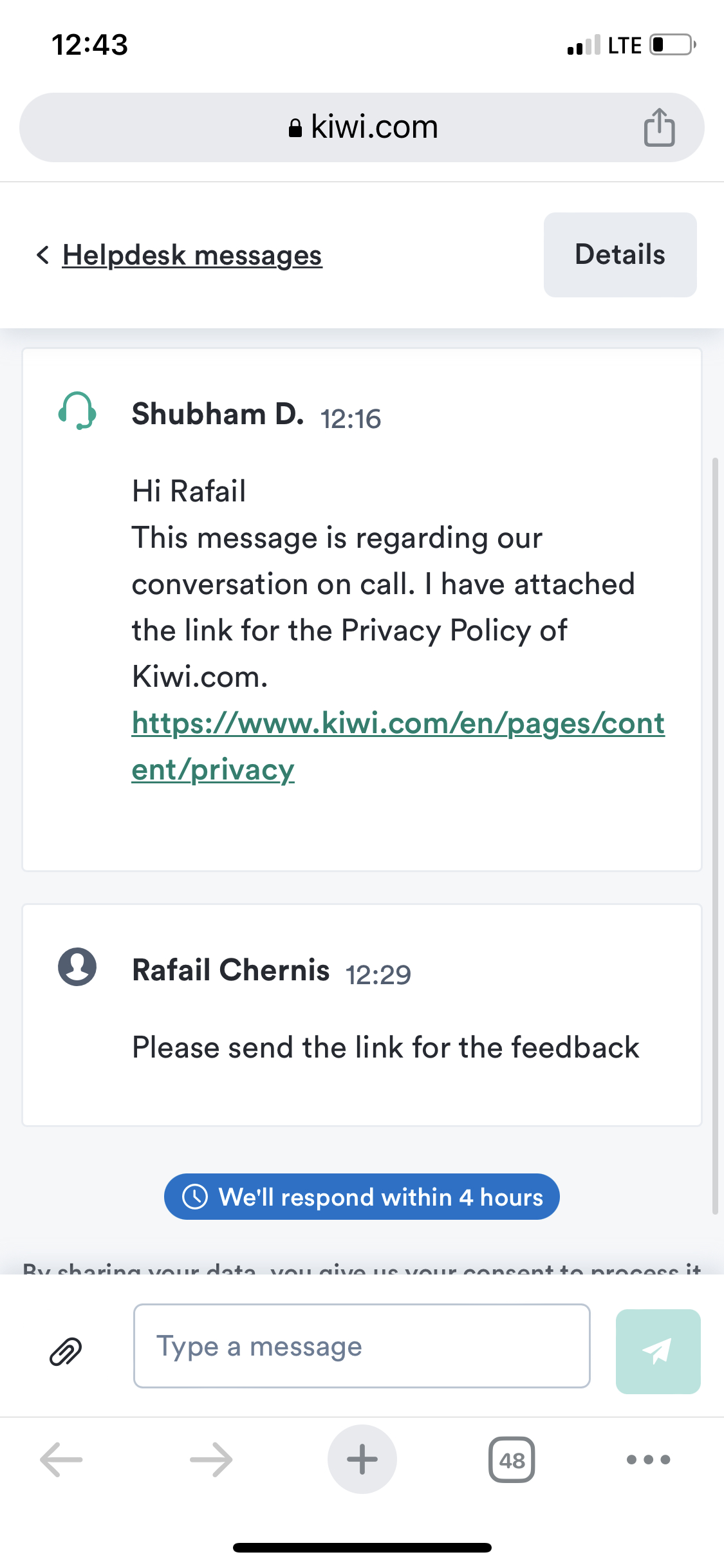On a mobile device using the Chrome browser or a similar interface, the user is navigating the Kiwi.com website. The screenshot displays a conversation with the Kiwi.com customer support team. The screen shows a back button labeled "Help Desk Messages," indicating that the user has entered a specific conversation. The chat features a message from customer support addressed to "Raphael," referencing an earlier phone conversation and including a link to the privacy policy. Raphael Chernus responds by requesting a link for feedback. Below this, there is an automated message stating that a response will be given within four hours. The chat message at the bottom is partially visible, mentioning something about sharing data. Additionally, the user has customized their browser interface, placing the search bar and tabs at the bottom of the screen instead of the top.